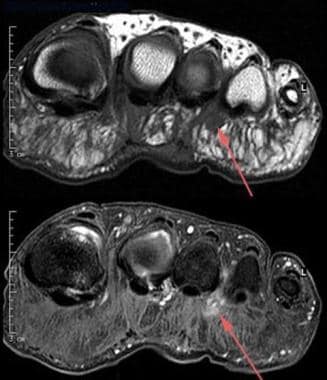This image comprises two MRI scans, shown one above the other against a black background, effectively stitched together. Both images feature the same elongated, vaguely blob-like structure reminiscent of a stubby caterpillar or worm, potentially representing a soft tissue cross-section. This structure is grayish-silver in color.

In the upper MRI scan, five circular voids or spots of varying darkness are visible within the tissue: a large dark spot on the far left, followed by three smaller spots of differing intensities (from dark to light), and concluding with a very tiny spot on the right. A red arrow points to the middle spot, one of the darker ones.

The lower MRI scan depicts a similar tissue structure, but in this instance, all the circular voids are uniformly dark. The identical red arrow again emphasizes the same central spot within the sequence of five voids. The consistent placement of the arrow in both scans suggests a focus on a particular feature or anomaly.